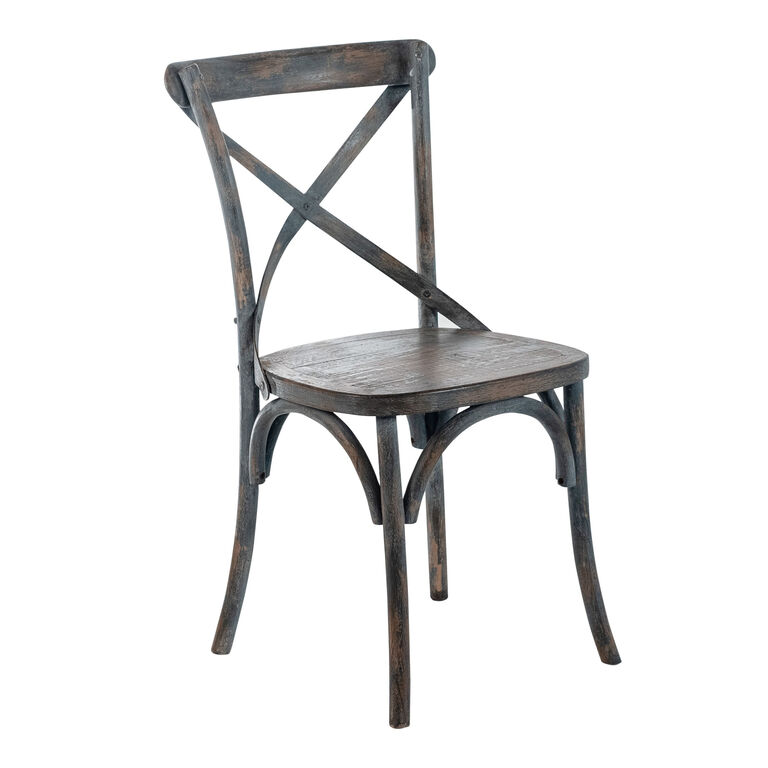This image, set against a plain white background, features a vintage-style dining room chair, combining both wood and wrought iron elements. The chair has four legs, each supported by a piece of wood forming an arch-shape, similar to an upside-down U, adding to the structural stability. The seat, made of dark walnut-stained wood, is a rounded square, giving it a classic look. The back of the chair is distinct, featuring two vertical posts with a wooden rectangle at the top, rounded at the corners. Across the back, two wooden straps form an X-shape, providing both support and aesthetic appeal. Additionally, there's a thin, oval-shaped piece of wood at the top of the backrest, also stained dark walnut. The metallic elements include two flat metal bands on the back that connect and support the chair, highlighting a blend of materials in its vintage design.